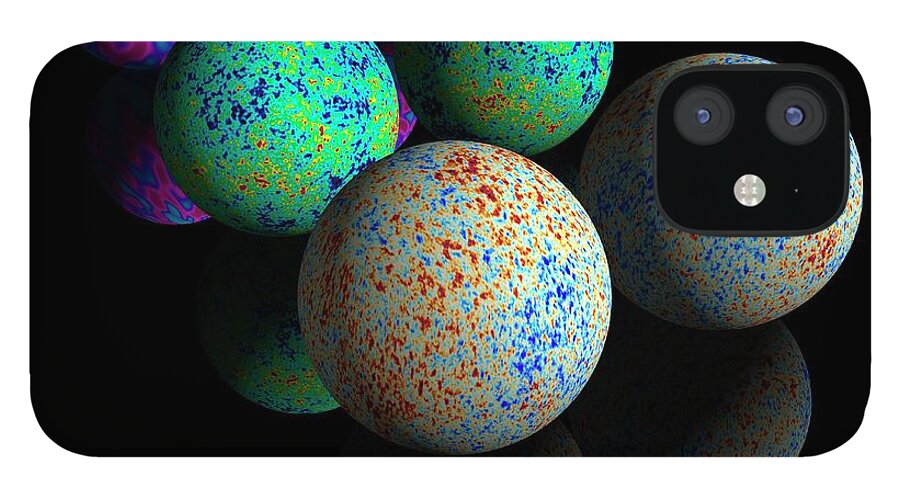This photo appears to be a computer-generated image depicting several colorful, speckled spheres that resemble globes or planets arranged on a small, square table. The spheres display an array of splatters in various colors. The most prominent sphere in the foreground features a white background with red, blue, and orange spots. To its right, another similar sphere can be seen, while further back on the left and top, there are a couple of spheres with green backgrounds and red and blue blotches. 

One sphere in the background is notably purple with blue patches. In the upper right-hand corner of the scene, there is a peculiar square object with rounded edges, resembling the back of a phone camera or possibly robotic eyes. This square has two circular shapes on top with glass in the center, evoking the appearance of a double-camera feature. The image is intricate and visually striking, blending elements of vibrant color patterns and enigmatic attachments, hinting at a possible automated or robotic theme.